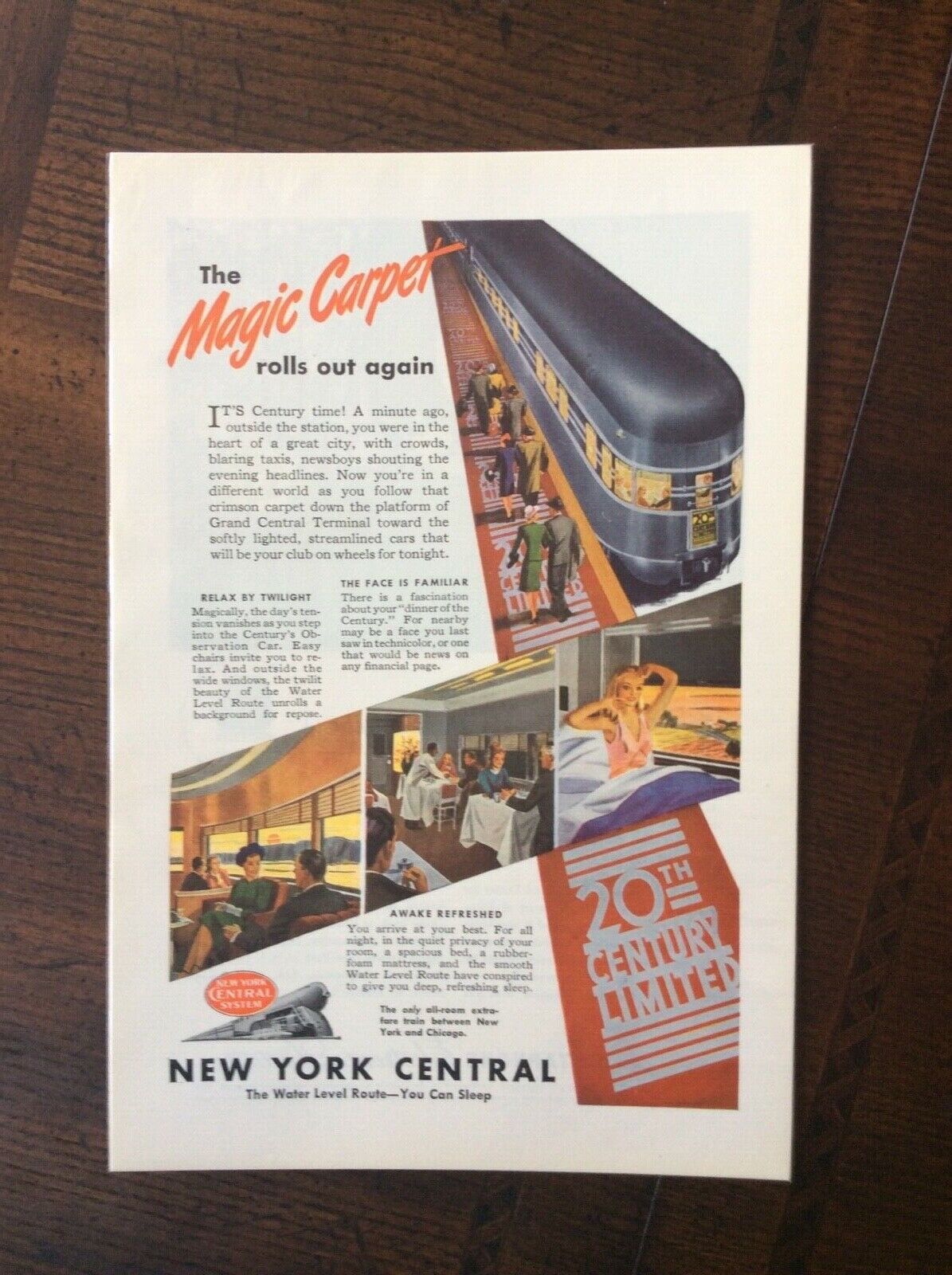The image depicts a page from a magazine or booklet, resting on a dark, wooden tabletop, possibly mahogany or walnut. The page, which has yellowed with age, prominently features an advertisement for the New York Central 20th Century Limited passenger service, with the bold headline "The Magic Carpet Rolls Out Again" at the top left. Dominating the right side of the page is an illustration of a streamlined, steel-gray train reminiscent of a mid-20th-century bullet train, situated on a platform where three well-dressed couples and a solitary man await. 

The bottom section of the advertisement includes three diagonally arranged parallelogram-shaped photographs stretching from the bottom left to the middle right. The first image shows a couple conversing on the train, the second captures a dining scene with passengers being served, and the third depicts a woman in her sleepwear stretching by an open window in her sleeping compartment. Directly below these images, more text appears, featuring a red banner with the words "20th Century Limited" and the bold label "New York Central." The entire page is rich with visual and textual details, reminiscent of a high-class promotional magazine spread from a bygone era.